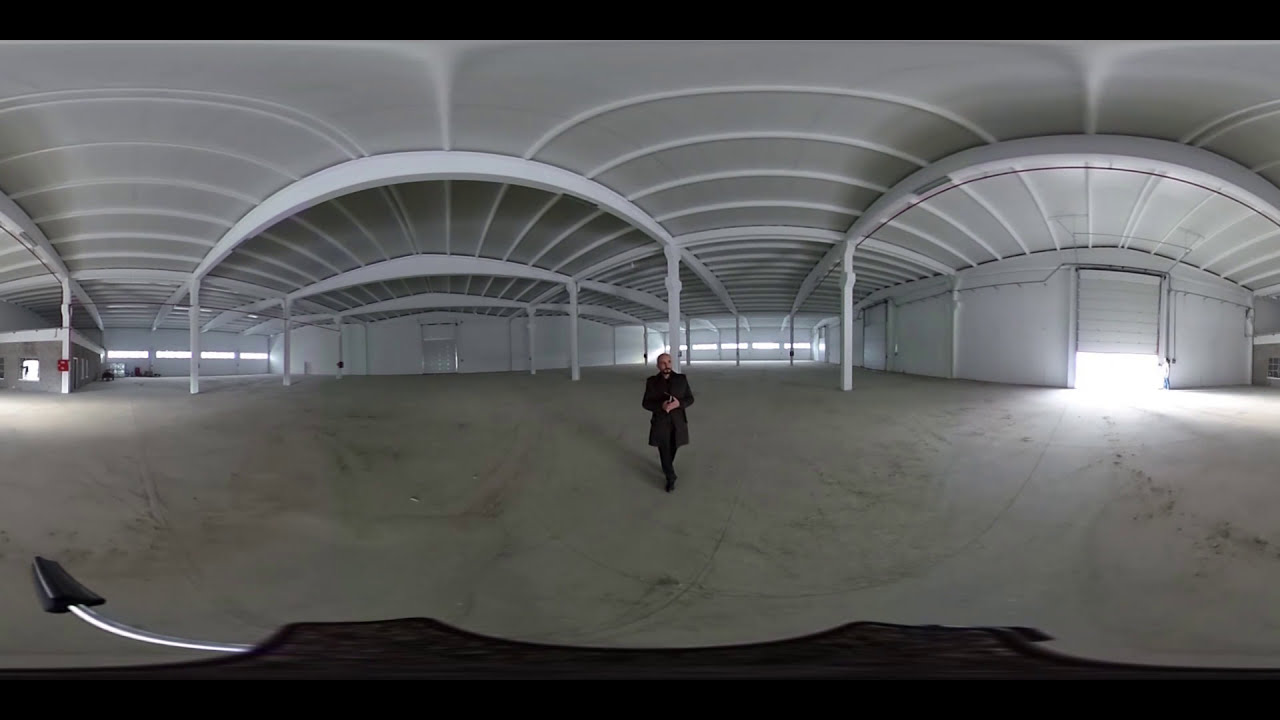This image portrays the interior of a vast, empty warehouse with an industrial aesthetic, captured with a fisheye or similarly distorting lens, creating a warped perspective. The warehouse exhibits a grey and white color scheme, with its expansive concrete floor and walls highlighted by curvature from the lens. Several white pillars punctuate the space, providing structural support. 

A bald man with a brown goatee is centrally positioned, walking towards the camera. He is dressed in a long black trench coat, black pants, black shoes, and a black shirt, which emphasizes his presence against the stark, minimalist background. 

Natural light floods in through a partially open shutter door, casting light onto the concrete floor and augmenting the sense of emptiness. Additional light enters through narrow windows along the sides of the building. The ceiling features steel girders and archways, which are also distorted into rounded shapes due to the lens effect, adding to the surreal quality of the scene. To the left, a white door adds another point of interest within the otherwise vast and open space.